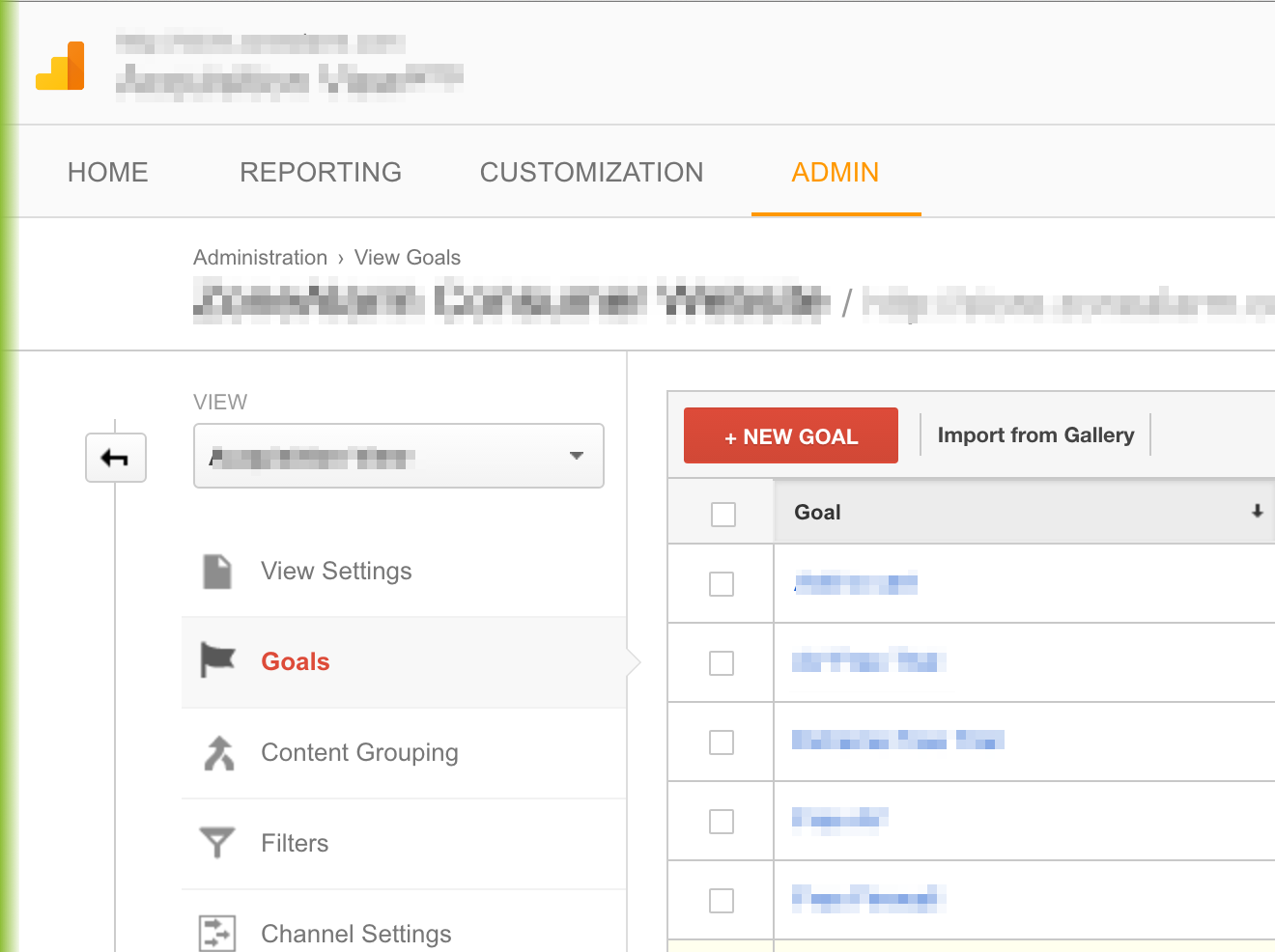The image showcases a web page or application interface, characterized by several sections and pixelated information that might be sensitive or personally identifiable. At the top of the page is an orange logo, accompanied by indistinct text that has been intentionally blurred. Beneath the logo, the interface features a navigation menu with the following options: Home, Reporting, Customization, and Admin. 

Directly below this menu, there is a header labeled "Administration - View Goals." Further down, another line of pixelated data appears, the contents of which are unclear. The left side of the page includes a vertical table with buttons labeled: View Settings, Goals, Content Grouping, Filters, and Channel Settings. 

To the right, another table features prominently, highlighting a red box or clickable button labeled "New Goal." Adjacent to this, there is another button that says "Import from Gallery." Below these buttons, a list is displayed with a header labeled "Goal," accompanied by a drop-down box; the remaining items on the list are also blurred out, maintaining the mysterious nature of the concealed information.